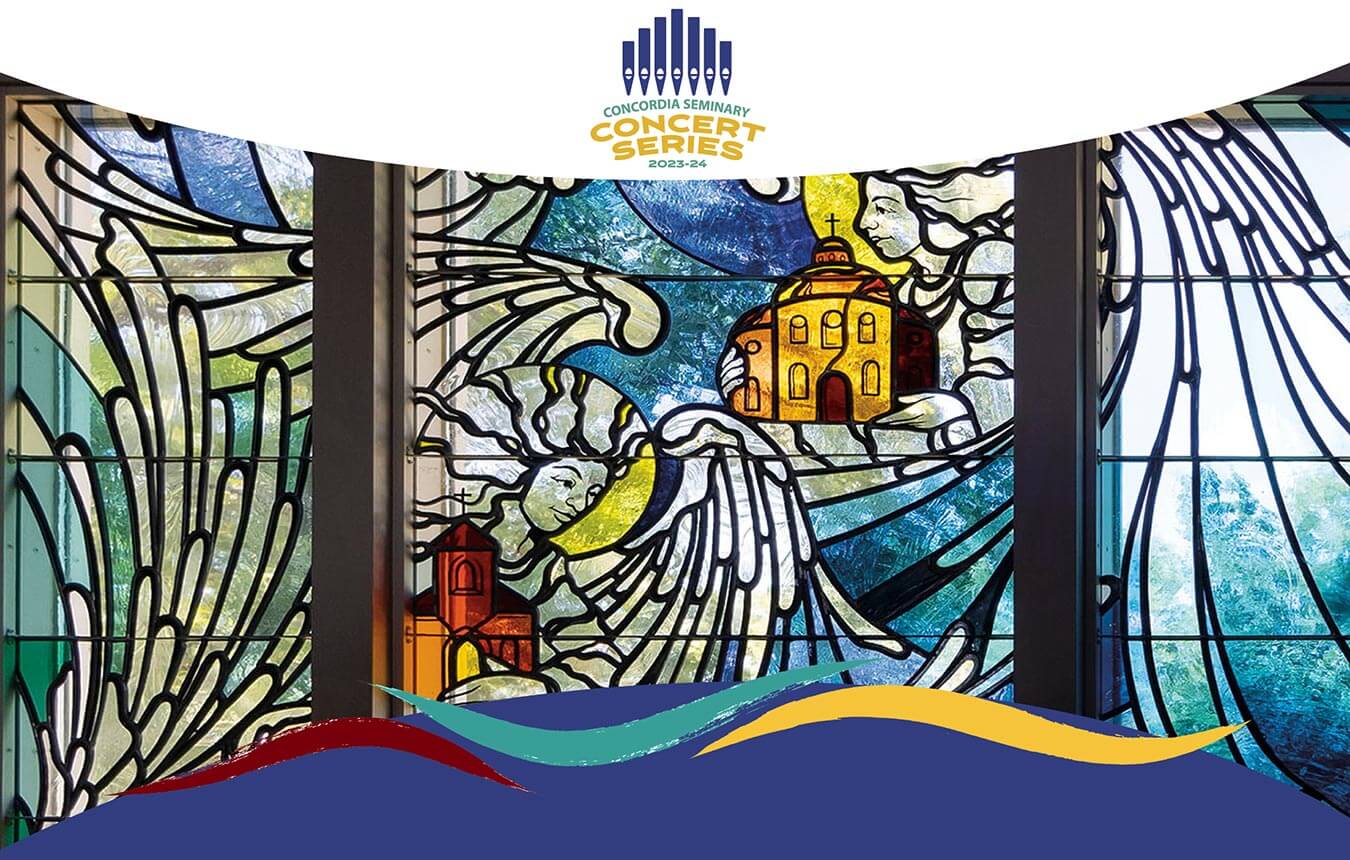The image is a wide poster for the Concordia Seminary Concert Series 2023-24. At the top, there's an arched, white background featuring seven blue organ pipes, which curve around blue and gold text that reads "Concordia Seminary Concert Series 2023-24." Beneath this text lies a vivid stained glass display divided into three main panels. 

The central panel showcases an angel, donned in white and black, with flowing hair and large wings, holding a cylindrical, yellow-orange church with a cross. To the right, another angel, also winged, cradles a red-orange triangular church with a cross. Both angels have yellow halos and are set against predominantly blue and green backgrounds. 

The side panels contain abstract designs, possibly depicting waves, leaves, or trees in blue, green, and white hues. The right side panel might show a clear sky with some trees. At the bottom of the stained glass is a semi-circular dark blue arch adorned with red, blue, and yellow squiggly lines, adding to the overall ornamental feel of the poster. The combination of rich colors and detailed imagery emphasizes its religious and artistic significance.